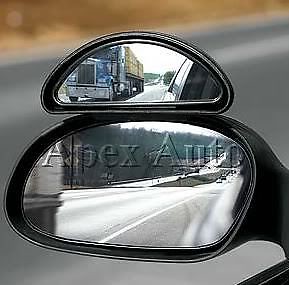This close-up photograph captures a side view mirror on a car, featuring two stacked mirrors—a larger, standard mirror on the bottom and a smaller, aftermarket blind spot mirror on top. The lower mirror reflects the view of a road with a portion of a truck's tail end and a mountainous background, possibly snowy or featuring a silver and white road. The upper domed mirror, affixed above the standard mirror, provides a wider angle, allowing the entire truck and some side panels of the car to be seen. This additional mirror, resembling a fisheye lens, offers a broader perspective, highlighting potential blind spots that the lower mirror might miss. The image includes a translucent "Apex Auto" watermark, positioned prominently. The backdrop is a road scene with some trees and minimal traffic, slightly blurred to emphasize the side view mirrors.